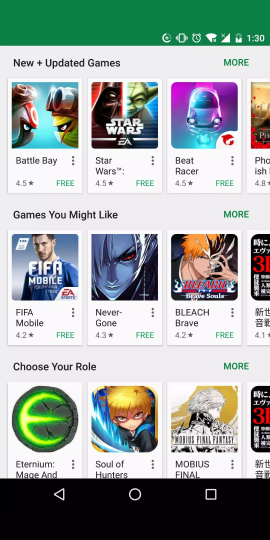The image appears to be a screenshot, likely from a mobile device, depicting a search interface for Google services. At the very top of the screen, there is a white area featuring the word "Google" in black text. To the left of "Google," there is a gray arrow pointing to the left, and to the right, there is an "x" symbol, which likely serves as a close button.

Beneath this header, there are several rows, each containing the icon of a magnifying glass followed by the name of a Google service. The services listed are:
- Google Pay
- Google Home
- Google Chat
- Google Photos
- Google Voice

Each row also includes a small arrow icon on the far right, pointing towards the northwest, indicating that these are links to individual sections or search results for each service.

At the bottom of the screenshot, there is a gray rectangle displaying an on-screen keyboard layout, similar to a computer keyboard, complete with all the letters. In the upper left corner of the keyboard, there is a blue circle with a right-pointing arrow, accompanied by the text "I," "2," and "U." On the right side of the keyboard, there is a microphone symbol, suggesting voice input capabilities.